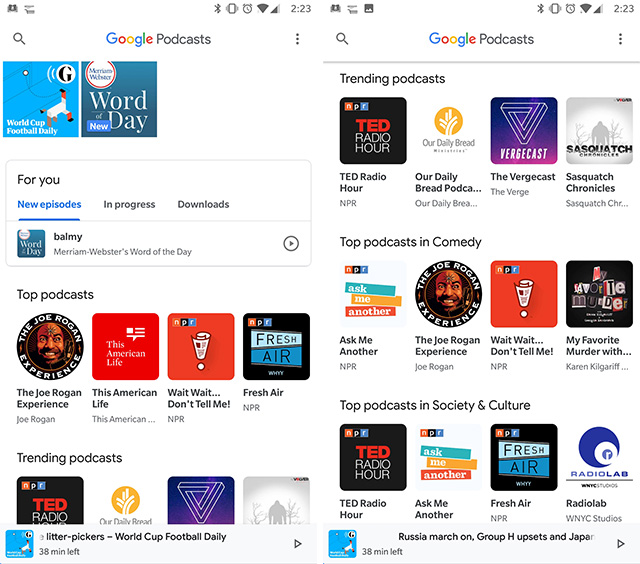The image displays a Google Podcasts interface rich with diverse podcast options. The central section prominently features a variety of popular shows: "TED Radio Hour," "The Daily Bread Podcast," "The Vergecast," and "Sasquatch Chronicles," among others. Comedy enthusiasts are invited to explore top choices such as "Ask Me Another," "The Joe Rogan Experience," "Wait Wait... Don't Tell Me," and "My Favorite Murder." For those interested in science and culture, highlighted podcasts include "TED Radio Hour," "Ask Me Another," "Fresh Air," and "Radiolab."

On the left side of the interface, users can find specific sections like "World Cup Football Daily" and "Word of the Day." A small box labeled "For You" presents new episodes, shows in progress, and downloads. This section features "Word of the Day: Balmy" by Merriam-Webster.

The platform also emphasizes top charts and trending podcasts, reiterating popular choices such as "The Joe Rogan Experience," "This American Life," "Wait Wait... Don't Tell Me," "Fresh Air," and "TED Radio Hour." Among trending podcasts, "Our Daily Bread," "The Vergecast," and "Sasquatch Chronicles" are notably featured.